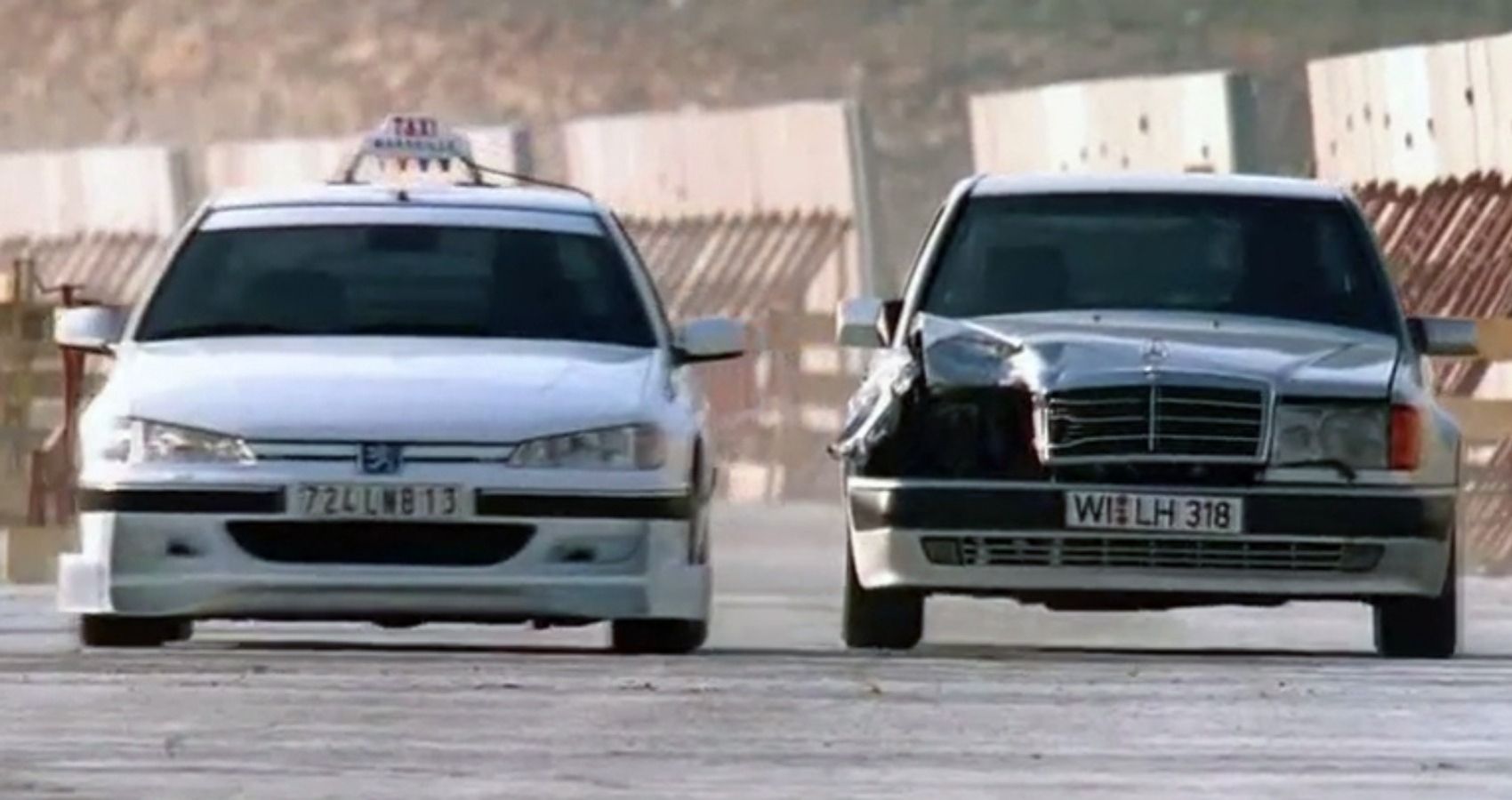The image depicts two cars positioned side by side, facing the camera. The car on the left is a white taxi in perfect condition, identifiable by a red taxi sign on its roof. The car on the right is a gray Mercedes with significant damage to its right-hand headlight and front bumper, suggesting it was involved in a recent collision. Both cars appear to be parked on a gray surface and fill the entire frame of the photo. Shadows inside the vehicles indicate there may be drivers sitting in them. In the background, a blurry hillside, brown terrain, and some white fences are visible, indicating the photo was taken outdoors, possibly around the late 1980s or 1990s due to the car styles and photo quality. The late-day sun casts long shadows, enhancing the natural light of the scene.